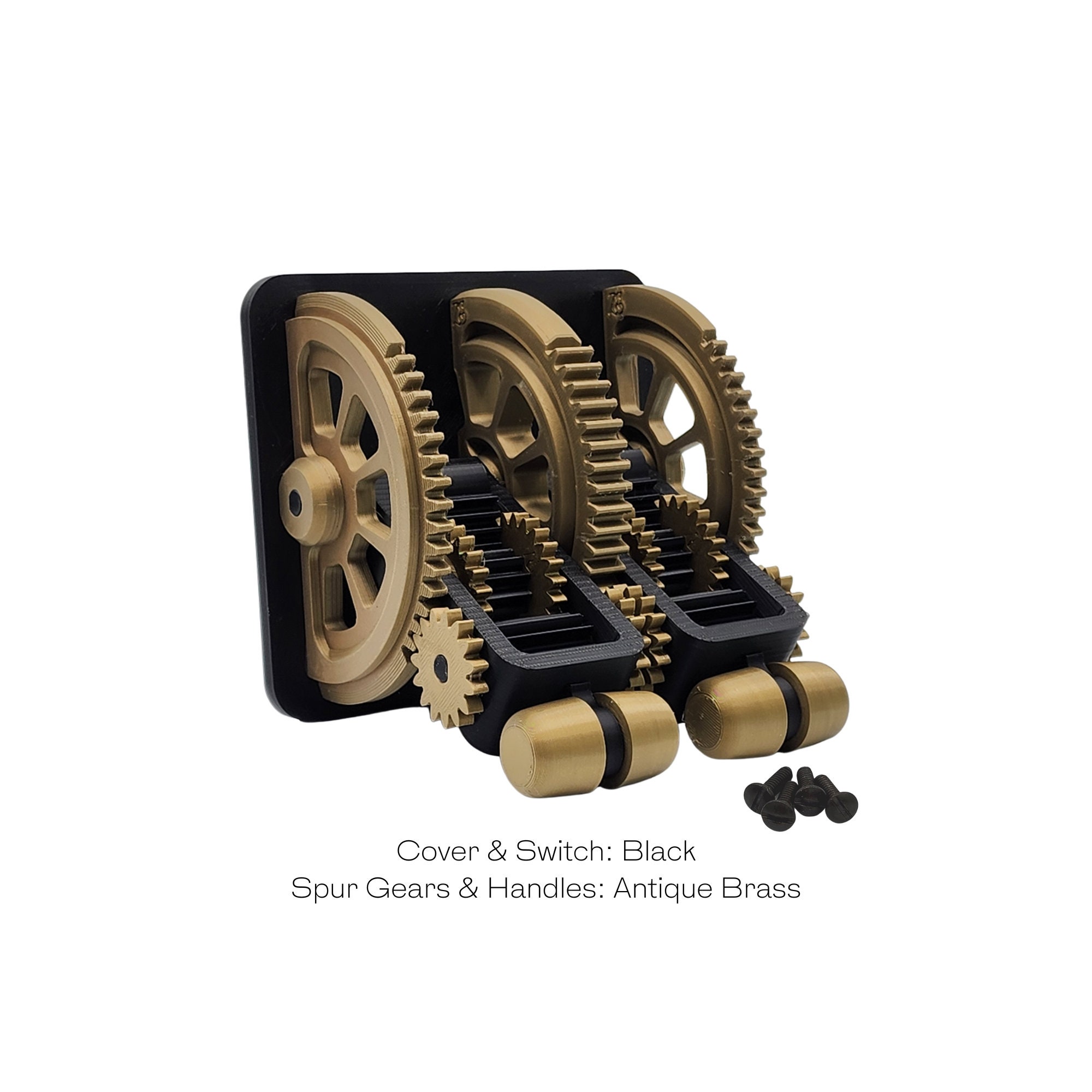The photograph showcases a steampunk-inspired device set against a white background. Central to the image are three large gears encircling a central stem, all rendered in an antique brass color. In front of these prominent gears, a series of smaller gears is intricately connected, including a notably tiny gear positioned near one of the larger ones. The ensemble of gears and handles is mounted on a black plate. Additional elements include two tan, cylindrical objects positioned in front of what seems to be a gear box container. Below the device, black text reads, "Cover and Switch: Black; Spur Gears and Handles: Antique Brass." Four small black screws are aligned to the right of this text. The combination of black and antique brass materials gives the device a striking aesthetic, reminiscent of steampunk design.